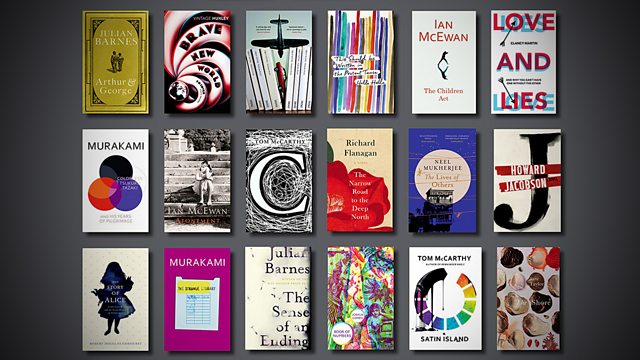The image showcases 18 books meticulously arranged in three rows of six on a gray background. The top row features Julian Barnes' "Arthur and George" with a yellow-green cover accented in black, "Brave New World" with a black background adorned with white and red swirls, an unreadable title featuring a blue cover with an airplane, a book with colorful stripes of purple, blue, red, brown, yellow, and more, Ian McEwan's "The Children Act" with a white cover and red lettering, and "Love and Lies" displaying a white background with blue and red text and arrows. The second row includes a Murakami book with black, blue, and red circles, a partially legible Ian McEwan book with a human figure on steps, Tom McCarthy's book with a giant black 'C' on a white cover adorned with scribbles, Richard Flanagan's book with a tan background and red floral-like patterns, one with a blue cover showing a moon and building, and Howard Jacobson's book marked by a giant black 'J' and red lines on a white background. The bottom row begins with a book featuring a black outline of a girl on a white cover, a Murakami book with a pink background and a white document, Julian Barnes' "The Sense of an Ending" in black text on a white cover, a tie-dye themed book with circles of unreadable white text amidst pinks, yellows, greens, and blues, Tom McCarthy's "Satin Island" exhibiting a color wheel and paint drips on a white cover, and finally, a book with color swatches of red, dark brown, white, and light brown on a gray background.